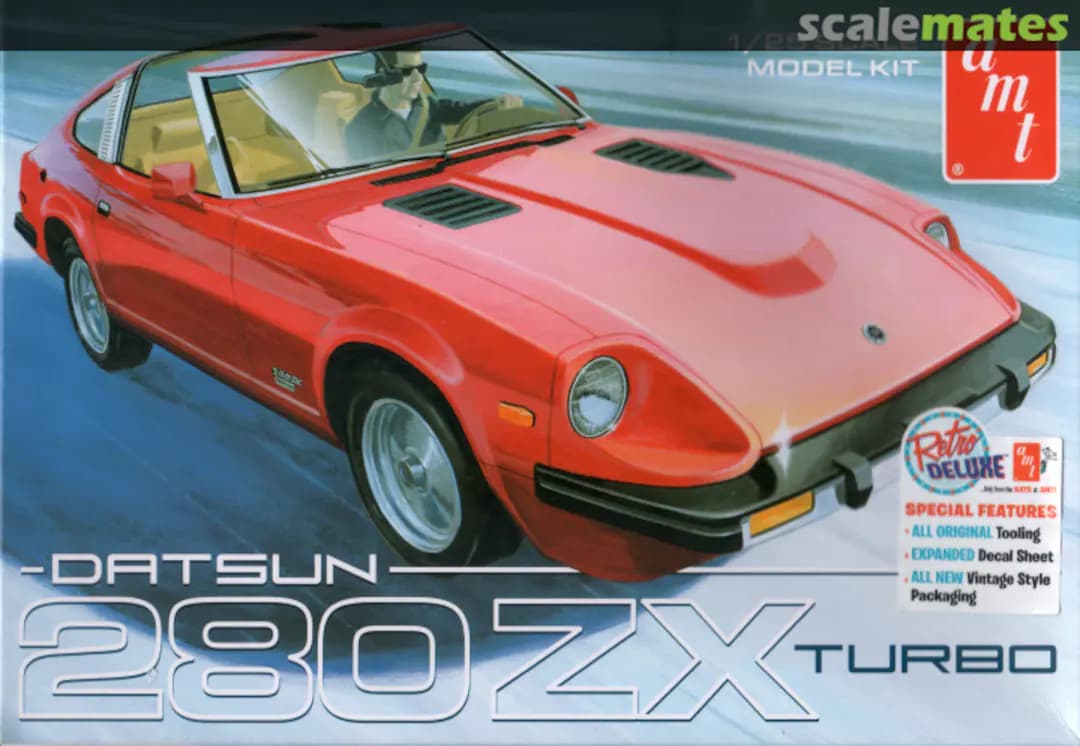This image is an advertisement for a ScaleMates Datsun 280ZX Turbo model kit, featuring a red, two-door sports car iconic of the 1970s. The car, depicted in a cartoon style, is driven by a man wearing sunglasses and a black jacket visible through the clear windshield, with a tan interior and black wheels. At the top, a black banner with the words "ScaleMates" in gray and green font sets the stage. White text in the upper left corner reads "model kit." An additional box in the top right contains "AMT" in white letters outlined in red. Along the bottom left, large white text states "Datsun 280ZX" beside a smaller "Turbo" in dark blue. The bottom right showcases a smaller ad with the phrases "Retro Deluxe," "special features," "all original tooling," "expanded decal sheet," and "all new vintage style packaging," with varied text colors of blue for emphasis.